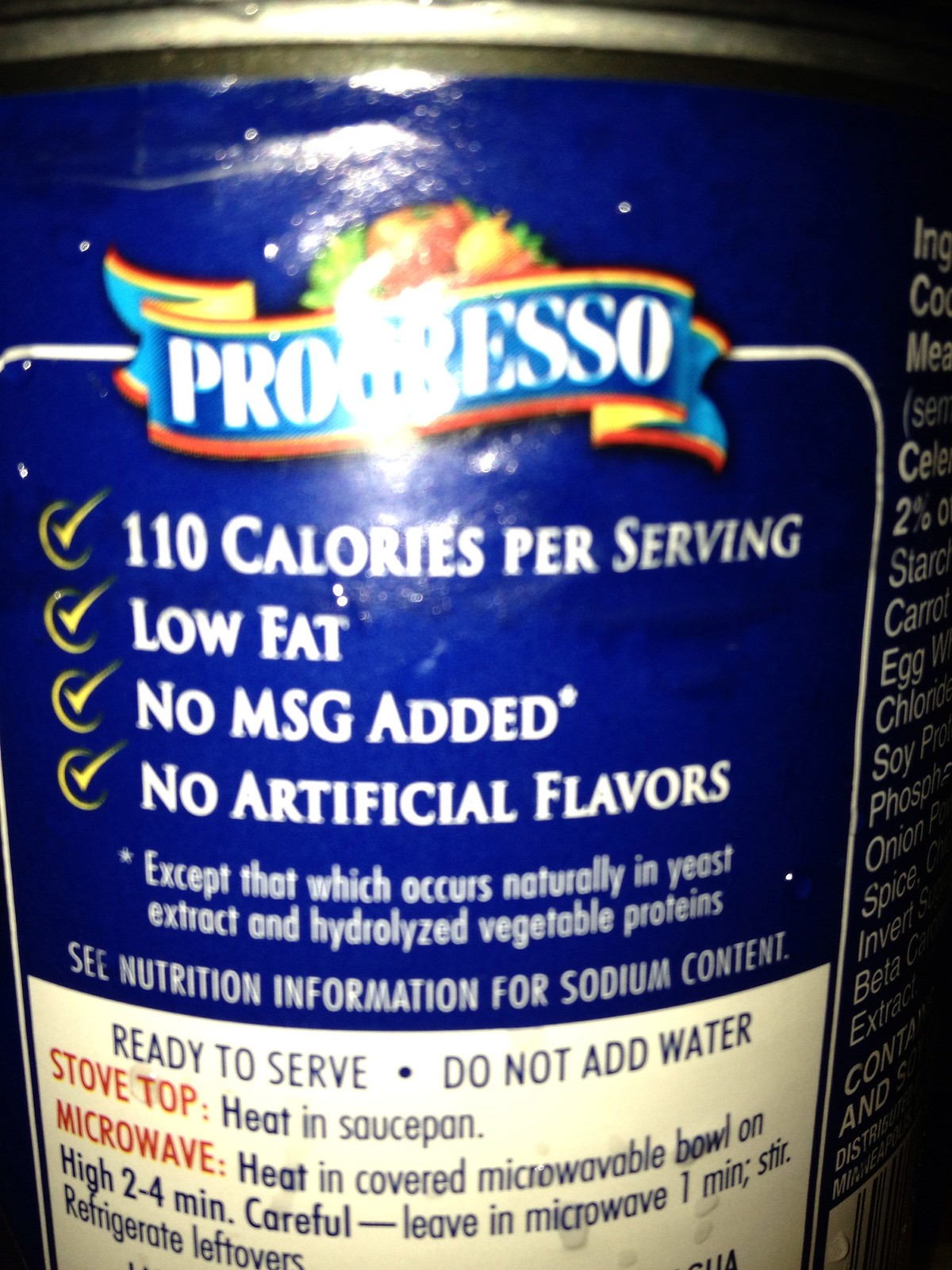This image features the side view of a Progresso soup can. The can has a prominent blue label with the brand name "Progresso" in white lettering, bordered by red and yellow stripes. The lighting causes a reflection on the can, making the text slightly difficult to read in certain areas. At the top, there is an image of various fruits and vegetables, signaling the presence of wholesome ingredients.

Below the Progresso logo, nutritional information is displayed, highlighting that the soup contains 110 calories per serving, is low in fat, and does not contain added MSG or artificial flavors—excluding naturally occurring substances in yeast extraction and hydrolyzed vegetable proteins. A note advises checking the nutrition information for sodium content.

The can also includes preparation instructions: it is ready to serve and should not have water added. Heating directions specify using a stove top by warming the soup in a saucepan, or a microwave by heating it in a covered microwave-safe bowl on high for two to four minutes. A cautionary note advises being careful when removing the heated soup from the microwave.